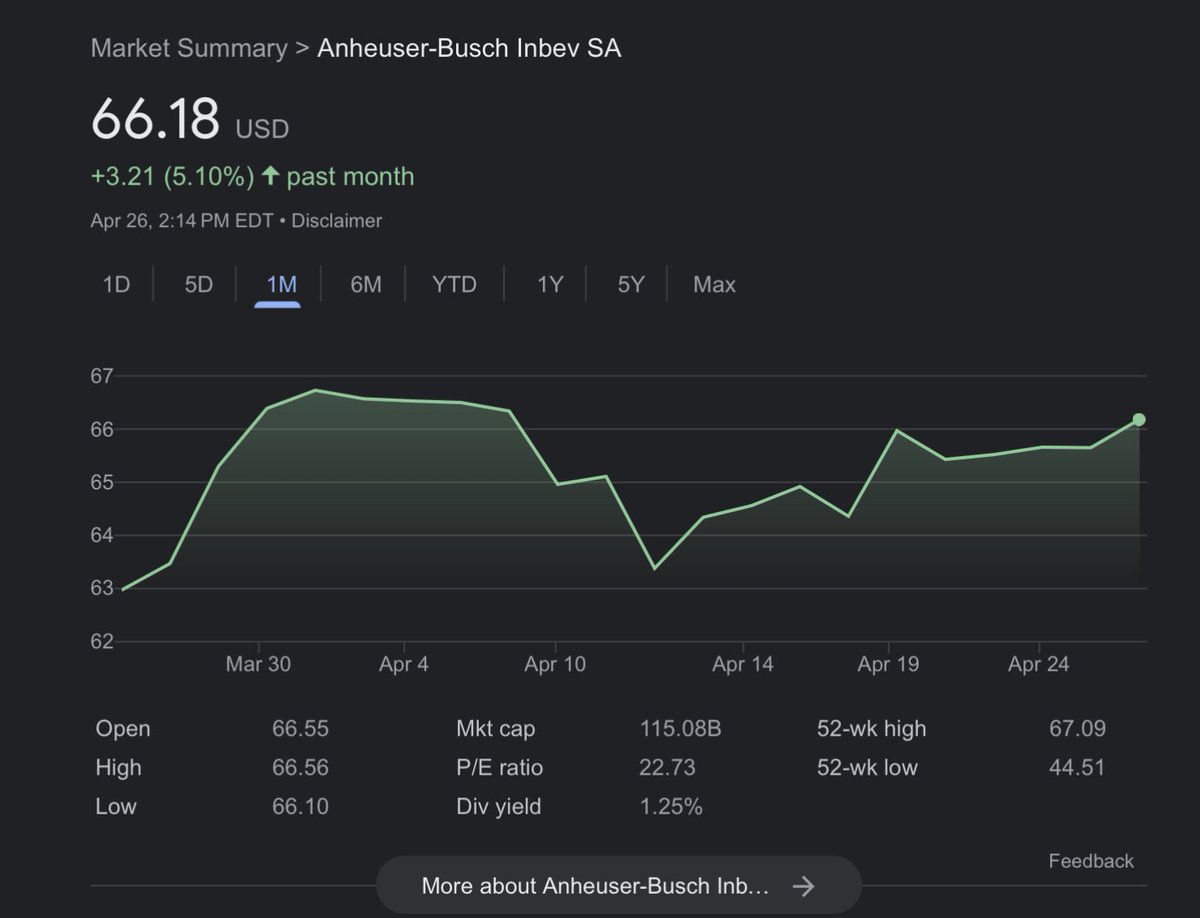In the image, the background features a gradient of dark gray shades. The top left corner prominently displays a microsummary of financial information. This section highlights "BulletinWebSA" with a current value of $66.18 USD, showcasing an increase of $3.21, which translates to a 5.10% growth. Below this, there is a row indicating various selectable time frames: 1 day, 5 days, 1 month, 6 months, Y2Z (Year to Date), 1 year, 5 years, and max. There is also a mention of "Apple 26, 2, 14 pound," though its context is unclear. Additionally, a shaded gray area provides more detailed insights, specifically related to feedback from "Sarah Bush."